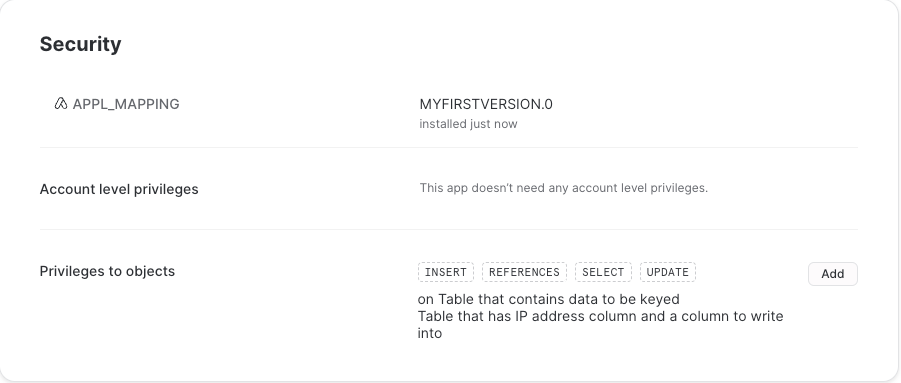The image depicts a section of a software interface focused on security settings, displayed on a white background. At the top, prominently in black lettering, is the word "SECURITY." Below this, an icon resembling the letter 'A' is labeled "APPL_MAPPING" in all capital letters. To the right, on the same row, the text "My first version 0.0" is visible, followed by the note "Installed just now."

A faint gray line separates this section from the next. The subsequent line contains the text "Account Level Privileges" in black print on the left, while the right side indicates, "This app doesn't need any account level privileges."

Further down, another faint gray line is followed by the label "Privileges to Objects" on the left. The right side features four horizontally aligned boxes with dotted borders. Each box contains a different label: "INSERT," "REFERENCES," "SELECT," and "UPDATE." To the far right of this lineup is a solid-bordered box labeled "ADD." The final section specifies, "On table that contains data to be keyed, table that has IP address column, and a column to write into."